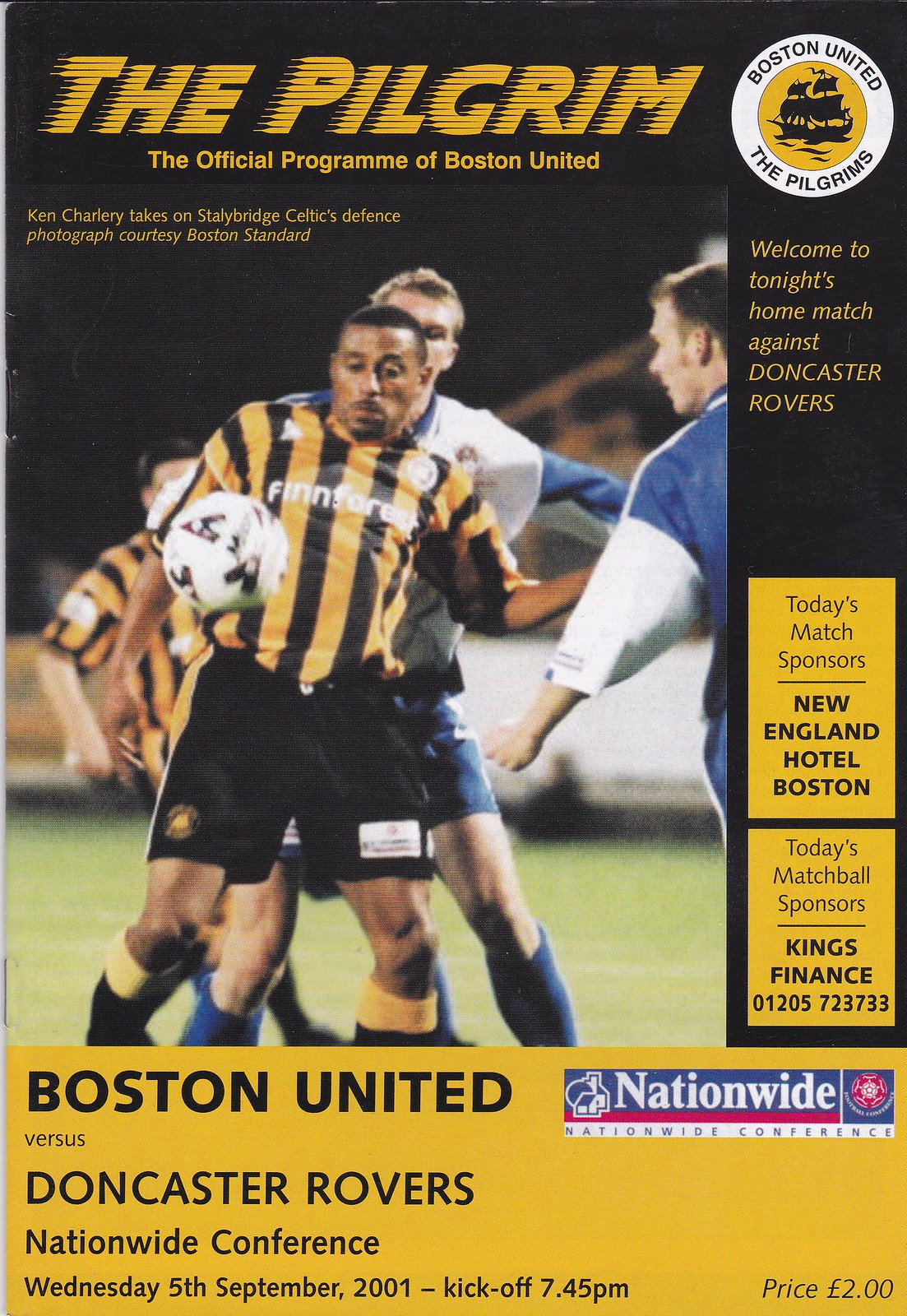The cover of "The Pilgrim," the official program of Boston United, features a dynamic and detailed design predominantly in black and bright yellow. At the very top, the title "The Pilgrim" is presented in bold yellow text, followed by the subtitle "The Official Program of Boston United." The left side of the cover showcases an intense photograph of a soccer match with four players, emphasizing the action on the field. In the foreground, a player in a yellow and black vertically striped jersey with black shorts is about to make contact with a soccer ball using his hip or waist, while being closely contested by players from the opposing team. One of the opponents is dressed in a white shirt, blue shorts, and blue socks. In the background, additional players add to the competitive atmosphere.

The bottom fourth of the cover features a yellow banner with important match details in black text, announcing the game between "Boston United vs. Doncaster Rovers" as part of the "Nationwide Conference" on "Wednesday 5th September 2001" with a kickoff time of "7:45pm." The price of the program, "£2.50," is noted in the bottom right corner of this banner. In the top right corner of the cover, a blue rectangle with white text advertises the "Nationwide Conference."

Additional annotations include "Welcome to tonight's home match against Doncaster Rovers" and mentions of today's match sponsors: "New England, Hotel Boston, King's Finance." Overall, the cover effectively captures the excitement of the match and provides key information for attendees.